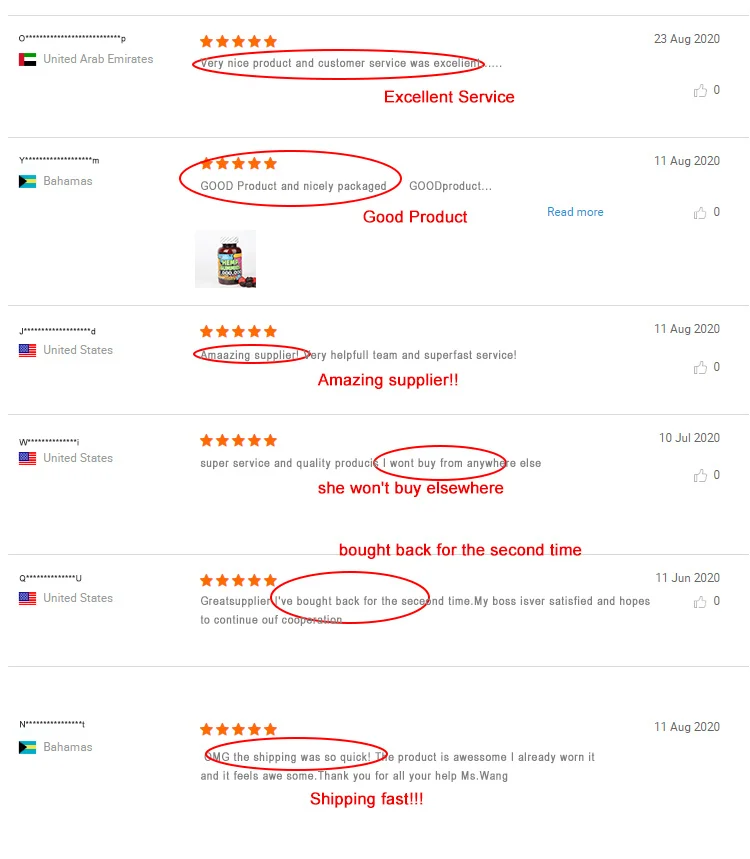The image depicts a review section from a website, primarily featuring a white background with black text. At the top left corner, there's a heading "United Arab Emirates" accompanied by a small UAE flag. Below this heading, the review displays five orange stars and the text "Very nice product and customer service was excellent," which is highlighted with a red circle.

To the right of this review, the phrase "Excellent service" appears in red text next to a thumbs-up icon, followed by "0 thumbs up."

Situated below and slightly to the right, another review features the Bahamas flag with the heading "Bahamas." The review states "Good product and nicely packaged," marred by another red circle, and awarded five stars. To the right of this, there's the text "Good product" with a clickable "Read more" link in blue.

Beneath the review from the Bahamas, there's an image of a bottle that resembles chewable gummy vitamins.

In total, six reviews are visible, originating from various countries including the United Arab Emirates, the Bahamas, and the United States.